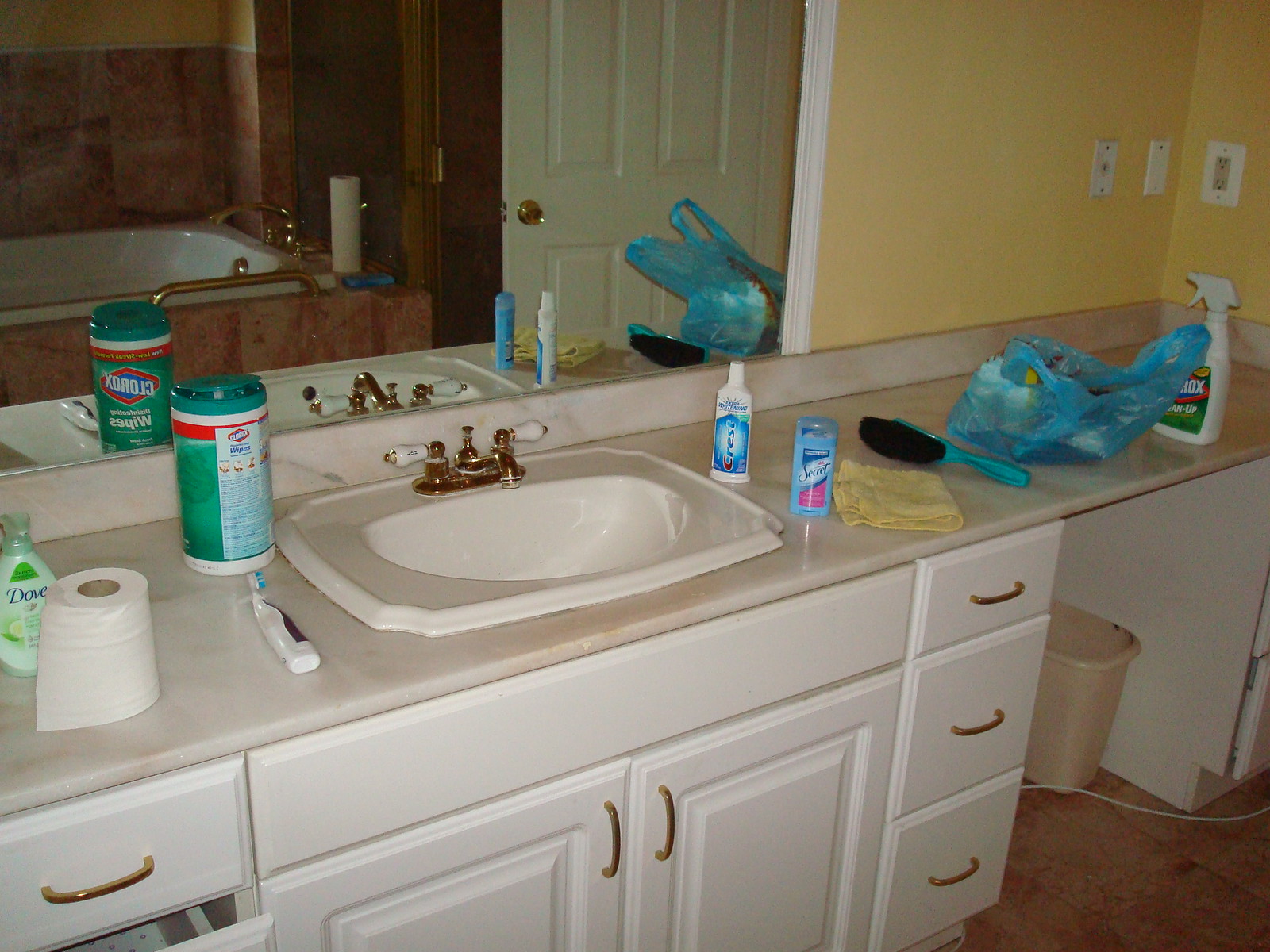This photograph showcases a meticulously detailed bathroom vanity set against vibrant yellow walls adorned with white wall outlets. The vanity features a sleek tan countertop, crowned with a pristine white sink and an elegant gold faucet complemented by white handles. Beneath the countertop are white cabinets, each accented with gold hardware.

The countertop is bustling with various items, reflecting everyday use. On the left side, a bottle of Clorox spray sits beside a white and green-labeled bottle featuring red and blue details. A blue plastic bag, seemingly containing assorted clothing, lies nearby. A blue hairbrush, a yellow washcloth, a blue deodorant stick, and a tube of Crest toothpaste add to the array of personal items.

On the right side of the sink, a white and blue toothbrush rests alongside a green-and-white package of Clorox wipes, accented with blue and red font. A half-used roll of toilet paper and a bottle of green Dove soap complete the assortment. Above the vanity, a mirror reflects the image of a bathtub, enclosed in a striking brownie-burgundy tiled surround with gold faucet hardware. A roll of paper towels is also subtly visible in the background, adding to the scene's realism and lived-in feel.